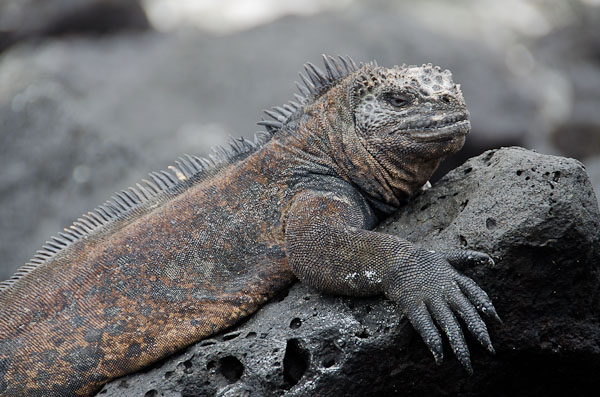This image is a striking, high-resolution photograph taken outdoors in bright daylight, featuring a close-up profile of a marine iguana. The iguana, captured in vivid live color, is sprawled lazily on a porous, volcanic black rock, almost hugging it. Its rigid and scaly skin exhibits an intriguing blend of reddish-brown and black mottling, blending seamlessly with the texture and color of the rock. 

The iguana's body stretches diagonally from the top of the photograph towards the lower left, drawing attention to its large, five-fingered black claw that prominently hangs off the edge of the rock. This claw is detailed, showing each digit and its formidable claws. The spiky ridge running from the iguana's head down to its tail accentuates its prehistoric and rugged appearance, with spines standing erect along its back.

The background is an artfully blurred out, muted gray rock that complements the primary subject, ensuring the iguana remains the focal point. The iguana's face, displaying a nonchalant and somewhat grumpy expression with slit eyes, conveys a sense of tranquility and indifference, as if it's basking in the sun and utterly unbothered by the world around it.